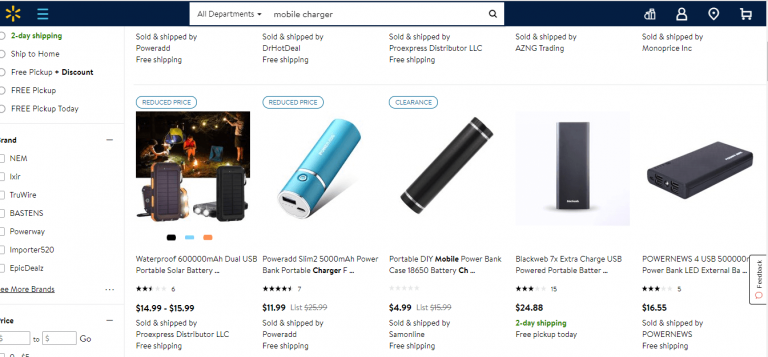The image displayed is a screenshot of the Walmart website. At the top left, there is a circular icon with yellow dashes. Adjacent to it is a search tab labeled "All Departments," and within the search field appears the text "mobile charger" accompanied by a gray magnifying glass icon.

Below the search bar are the search results starting with the first item: a waterproof, portable solar battery pack, featuring an image of several battery packs. This product has received a rating of 2.5 stars based on 6 reviews and is priced between $14.99 and $15.99. It is sold and shipped by Pro Express Distributor LLC, and it includes the option of free shipping.

The second listed item is the PowerAdd Slim 2 5000mAh Power Bank Portable Charger in blue, characterized by a compact design with a small port. It has earned a 4.5-star rating based on 7 reviews, and is offered at $11.99, reduced from a list price of $25.99.

Next, there is the Portable DIY Mobile Power Bank Case, available for $4.99 with a previous list price of $15.99.

The following product is the BlackWeb 7x Extra Charge USB Portable Battery, shown in black. This item has a 3-star rating from 15 reviews and is priced at $24.88. It offers 2-day shipping or the option for free pickup today.

On the left side of the page, a variety of filters are available to refine the search, including options such as 2-Day Shipping, Ship to Home, Free Pickup Plus Discount, Free Pickup, and Free Pickup Today. Users can also enter a specific price range and utilize numerous additional filters to customize their search.